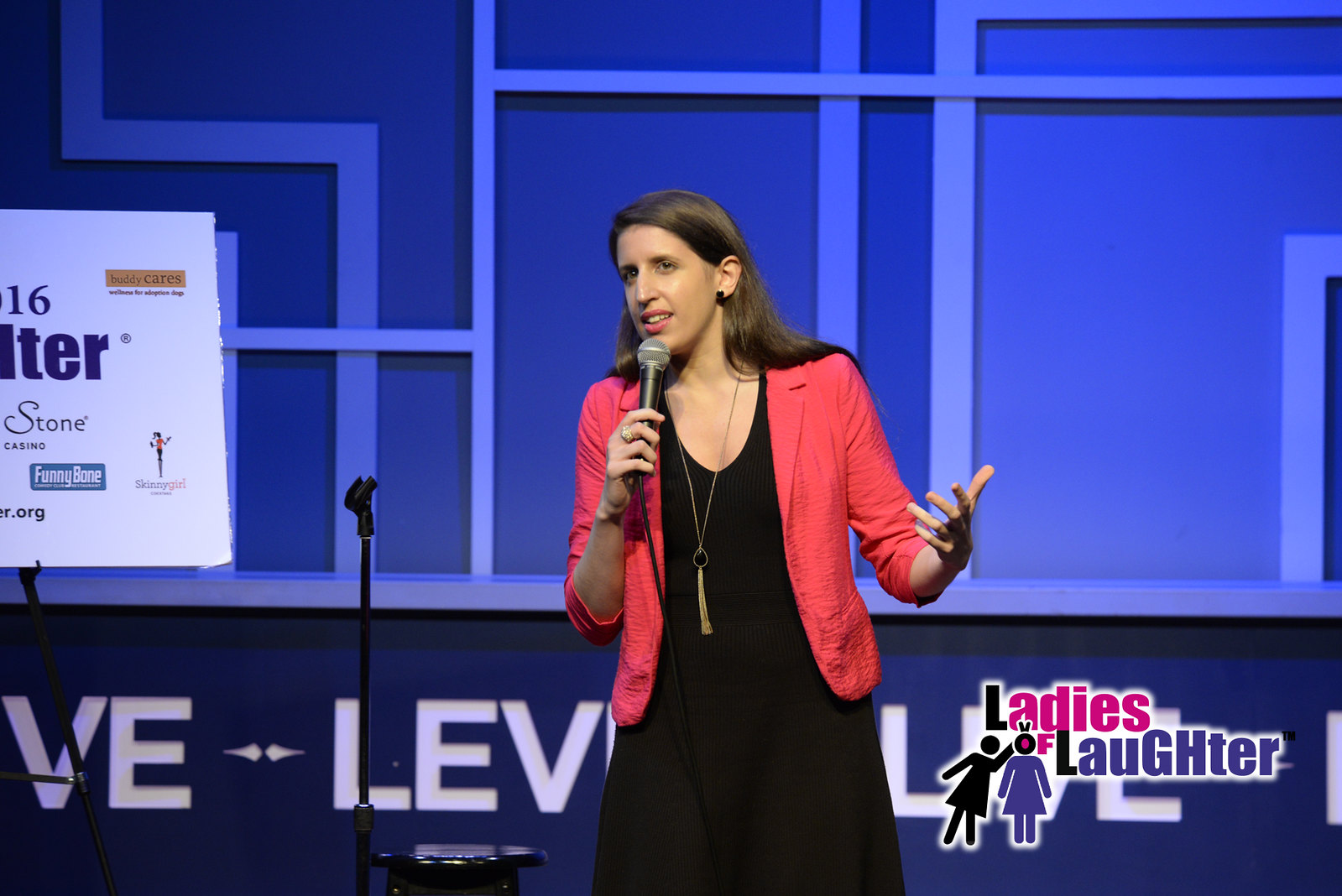The photo captures a young woman standing on a stage, likely performing as a comedian at a "Ladies of Laughter" event. She has long brown hair and is elegantly dressed in a long black dress paired with a pinkish-red blazer. A long gold necklace hangs around her neck. She is holding a microphone, speaking to the audience against a blue backdrop. On the left side of the image, there is a partially visible white poster featuring multiple logos and names, including "Funny Bone," "Bunny Cares," and "Skinny Girl." The lower right-hand corner of the photograph also features the "Ladies of Laughter" logo accompanied by two cartoonish graphics of women, with one playfully giving bunny ears to the other.